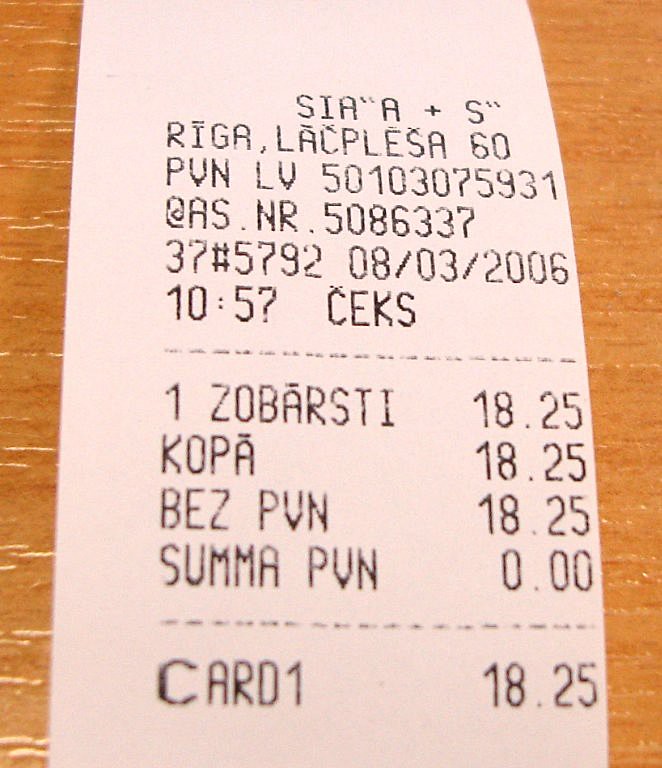A detailed caption for the image:

"The image showcases a white receipt with black text, placed on a tan surface. The receipt is printed in a foreign language and features several detailed entries and numbers. At the very top, there is text that appears as 'SIAA + SRIGR, LACPLESAS 60 PVNLV,' followed by a series of numbers. Below this, another line reads 'AS. NR' followed by another string of numbers, specifically '37-5792.' The date on the receipt is 'August 3rd, 2006,' with a time indicated as '10..5' with a question mark symbol and 'CEKS.' Further down, the receipt lists items such as '1 ZOBARSTI 18.25,' 'KOPA 18.25,' 'BEZPVN 18.25,' and 'SUMMAPVN 0.00,' concluding with 'card 1 18.25.'